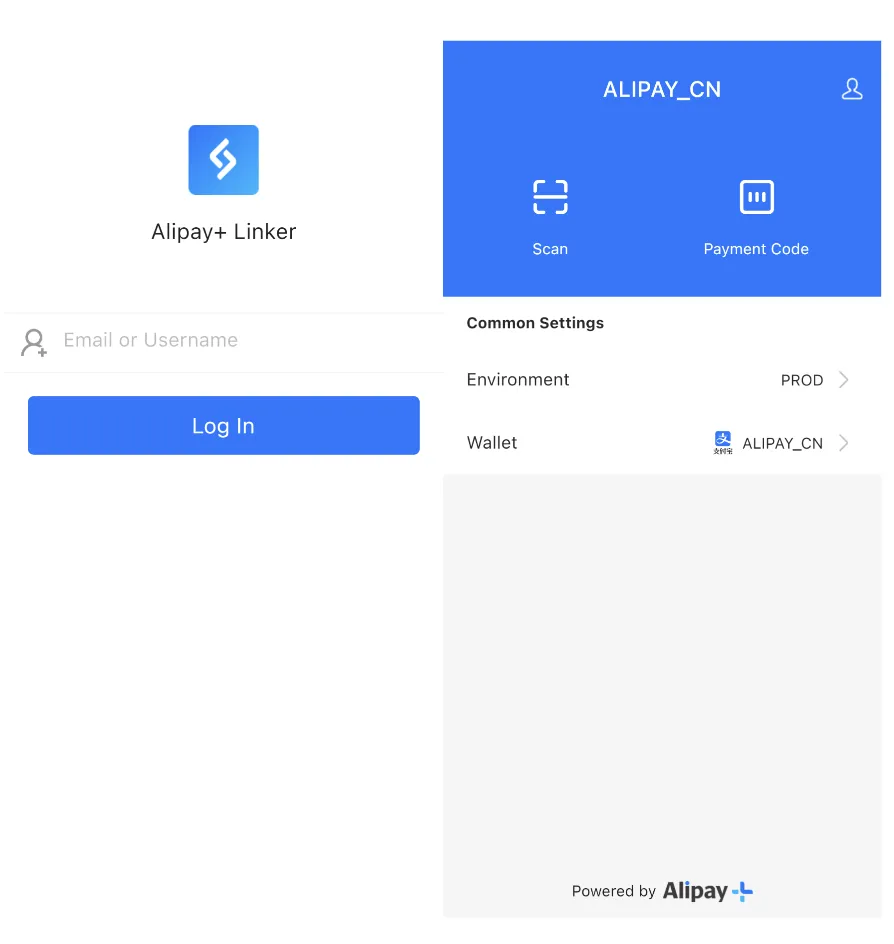The image appears to be a screenshot capturing two different pages of the same application. On the left page, the header reads "Alipay Plus Linker." Below the header, there is a text input field labeled "Email or Username," and beneath this field, there is a prominent blue button labeled "Login."

The right page's header displays "Alipay_CN" with two icons on either side: a "Scan" option on the left and a "Payment Code" option on the right. Directly underneath the header, it reads "Common Settings," followed by "Environment: prod" and "Wallet: Alipay_CN.” At the very bottom of the screen, there is text stating "Powered by Alipay," accompanied by a blue checkmark logo.